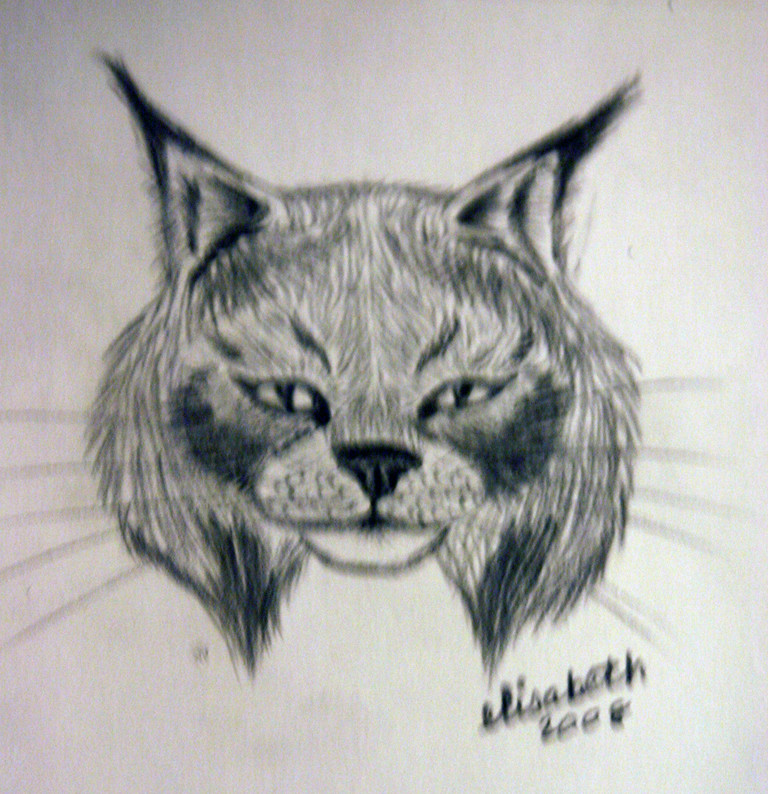The image is a hand-drawn, monochromatic illustration of a cat's face, created using a pencil or black pen on white paper. The cat's visage is detailed and symmetrical, featuring pointed ears with distinctive black tips and thin tufts of fur extending from the peaks. The cat's eyes are almond-shaped with vertical pupils, giving it a serious, almost piercing look as they gaze directly at the viewer. Long, shaggily styled fur frames the face, angling down beneath the rounded chin. The cat's nose is small and triangular with prominent whiskers fanning out from either side. Although the image is slightly blurry, it remains legible and is signed by the artist, Elizabeth, with the date 2008 in cursive at the bottom right corner.